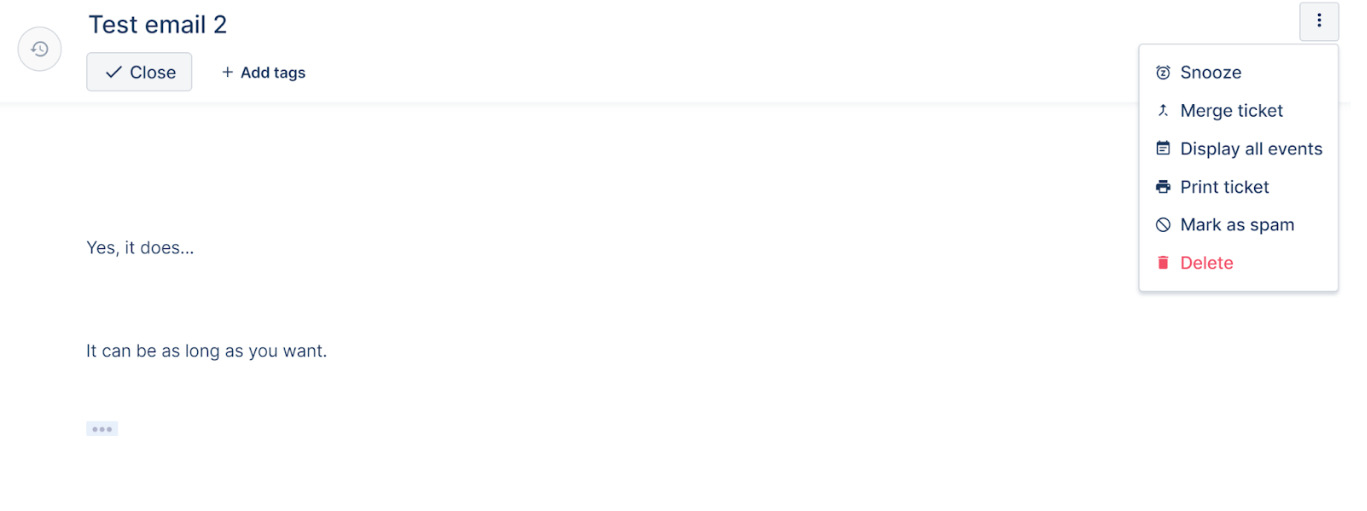The image depicts a plain and generic web page interface, presumably viewed on a computer. Dominating the top of the screen is the label "test email 2" rendered in bold black text. Just below this label lies a gray button featuring a check mark and labeled "close." Adjacent to it is a plus sign with the text "Add tags."

A gray horizontal bar separates this section from the next, which contains the text "Yes it does..." in black print. Further below, another line reads "It can be as long as you want." Positioned beneath this text is a very light gray square containing three faint dots, providing a subtle visual element.

In the upper right-hand corner, there's a gray box with three vertical dots. Below this box, a larger white box presents several options: "Snooze," "Merge ticket," "Display all events," "Print ticket," and "Mark as spam." The final option in this list is "Delete," distinguished by its red text and accompanied by a trash can icon.

Apart from these elements, the webpage is devoid of other content, maintaining a simple and unadorned appearance.